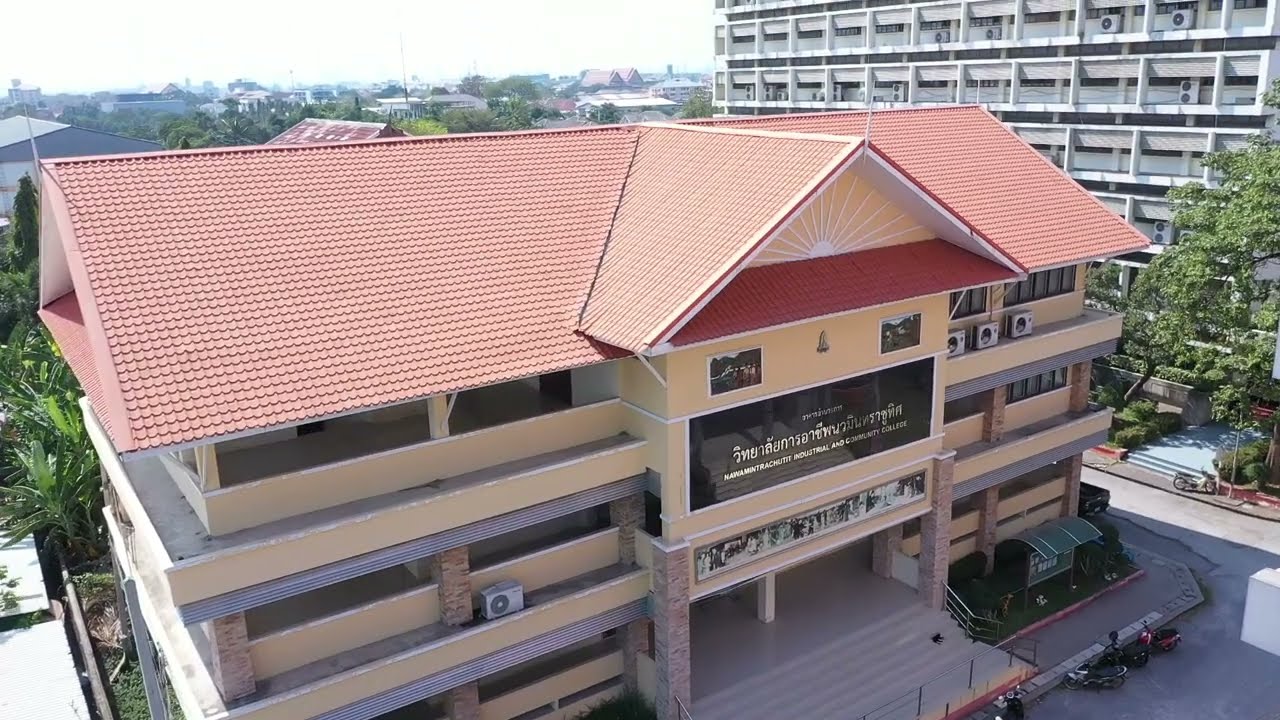The image showcases a high-angle view of a multi-storied industrial and community college, possibly located in Southeast Asia, suggested by the Indonesian-like script on the large black reflective sign on the building's facade. The structure is predominantly cream-colored with a distinct terracotta-tiled roof, featuring a central hipped triangle design. The building, composed of beige stone, includes multiple air conditioning units and a wide entrance flanked by a notice board. In the lower part of the image, there are several parked scooters or mopeds, emphasizing the urban setting. The environment is lush with tropical vegetation, including palm trees, blending seamlessly with other buildings around. In the background, a tall, multi-story apartment or hotel building with balconies, painted white, can be seen amidst the cloudy yet bright sky, reinforcing the image's urban and verdant scene.